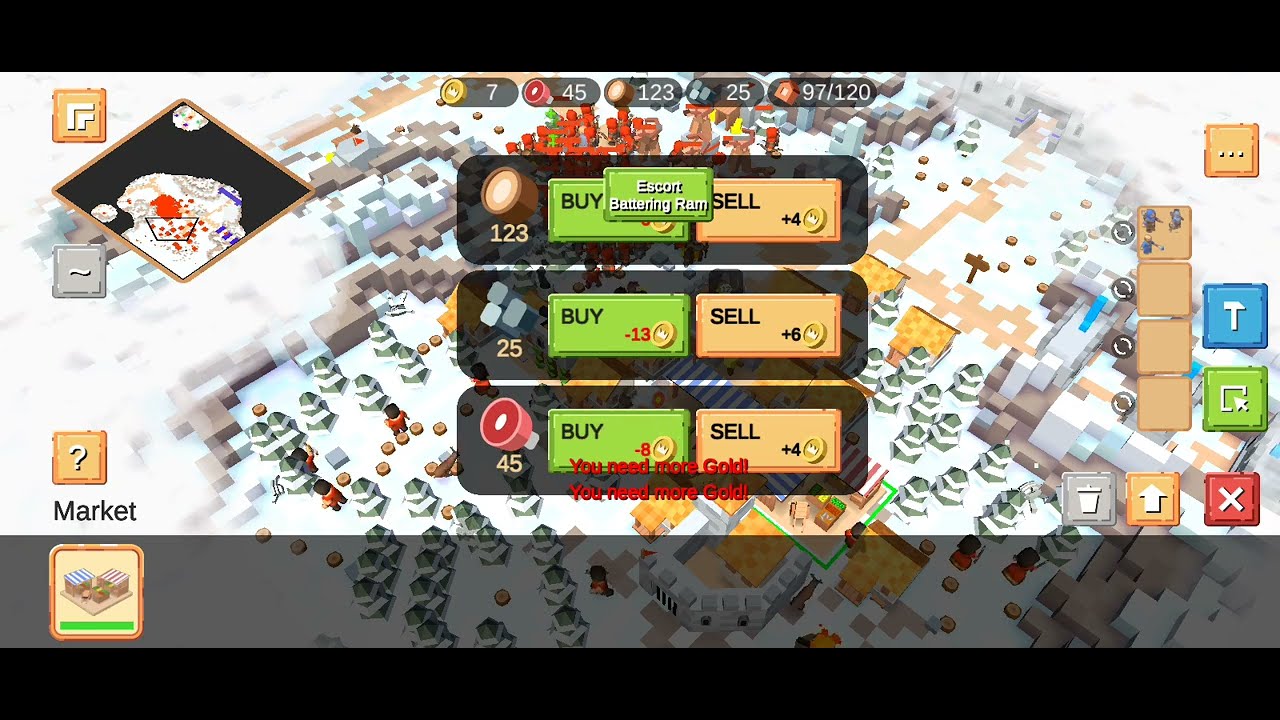The image appears to be a screenshot from a video game, likely a real-time strategy or base-building game, showcasing an aerial view of a village set in a snowy landscape. The scene features crudely constructed block houses interspersed with blocky green and white trees. At the very top of the screen, there are various icons indicating in-game resources: a coin icon displaying 146, a red meat icon with the number 5, a log icon showing 6, and a stone icon with 10. The left-hand side of the screen features a minimap, showing a broader view of the game's terrain.

In the center of the image, prominent menus are visible, providing options to buy and sell items. These menus display current resources: six logs, ten stones, and five meats, along with buttons to buy and sell these items. The word "Market" is visible at the lower left corner, suggesting the active menu's purpose. On the right side of the interface, various control icons are present, including a blue square with a white hammer for building, a stone pick, a mouse cursor, a red X, and an upward-pointing arrow.

The interface design and the visible statistics indicate that the player is managing resources and constructing buildings within the game environment.